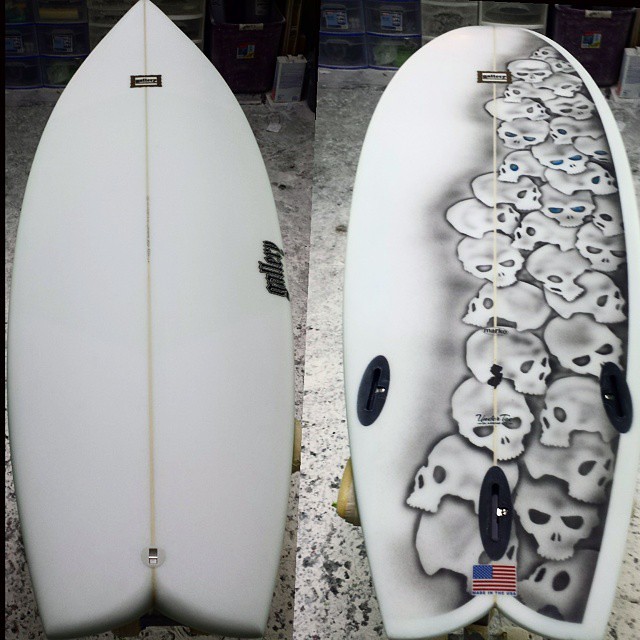The image displays a short surfboard shown from both sides, divided by a vertical line. On the left, the surfboard is plain white with a light beige line running down its center and a logo situated towards the middle right side. The right side of the split image reveals the flip side of the surfboard, which is richly adorned with overlapping white and gray skulls, primarily along the right side. Towards the base of the surfboard on this side, a small American flag is visible. The board rests on a textured cement or granite surface, and the background is cluttered with stacked plastic bins.